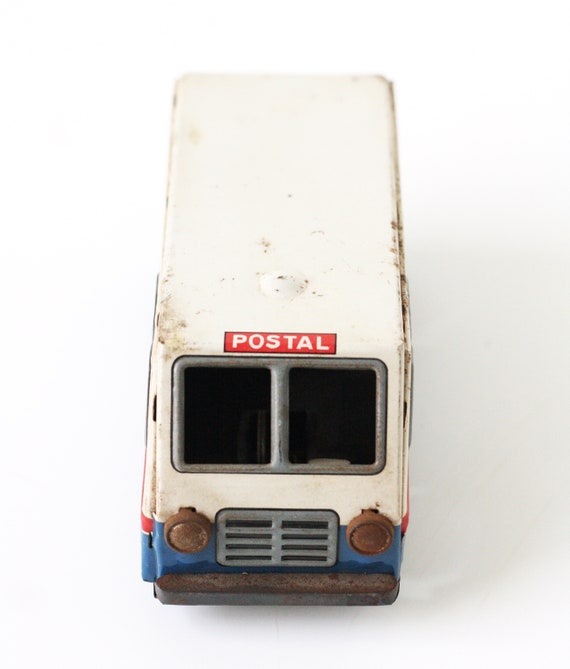The image depicts a weathered and corroded child's toy postal truck viewed from the front. This metal vehicle, likely once part of a child's fleet of toy cars, shows significant signs of aging and rust, especially on the headlights and bumper. The once shiny chrome headlights have turned dark brown with rust, and the front grille, situated between the two headlights, is gray. Above the windshield, the word "POSTAL" is prominently displayed in red lettering within a white rectangular block, bordered by a red outline and underlined by a dark blue stripe. The toy truck is primarily white with the top section painted white and the bottom band in dark blue. The vehicle's paint has chipped in several areas, evident of extensive play or perhaps having spent time buried underground. The light gray background contrasts slightly with the toy, which casts a shallow shadow, emphasizing its three-dimensional nature.